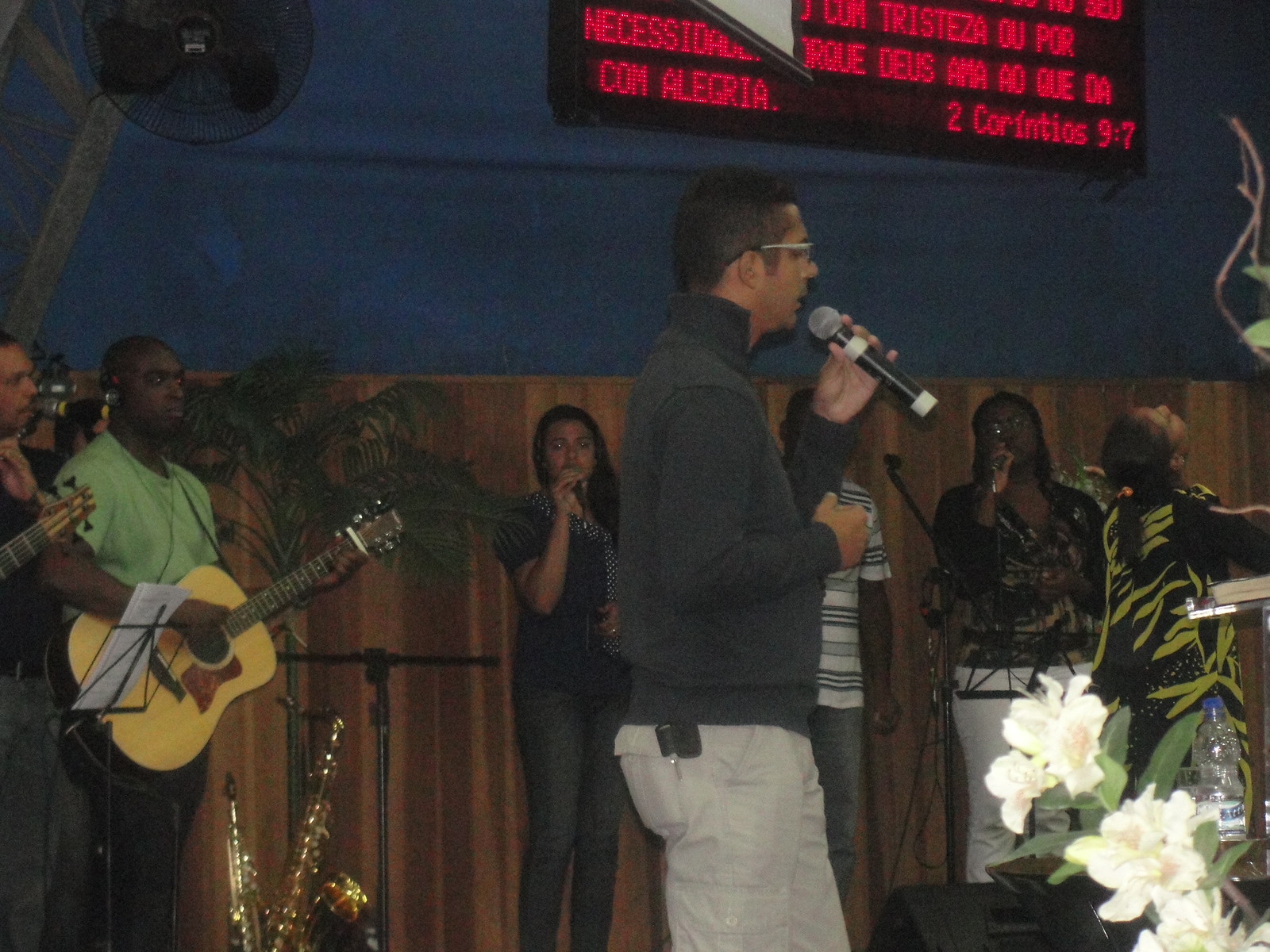In this horizontal rectangular image, a lively and youthful band is performing at what appears to be a church event. At the forefront stands a young man, possibly of Dominican descent, wearing a brown jacket and khaki pants. He faces to the right side, holding a microphone to his mouth, suggesting he is singing. The dim lighting casts a dark ambiance over the scene, but the blue wall and wood paneling in the background provide some contrast. The background hosts several performers: a guitarist, at least three backup singers with microphones, and other musicians, including someone playing a saxophone. A distinct feature above the performers is a sign with the words "Algeria" and a board referencing "Second Corinthians 9-7" in a different language, indicating this is indeed a church setting. Bright white flowers with green leaves, likely lilies, are visible in the lower right corner, adding a touch of elegance to the scene. The band members, aged between roughly 18 to 25, are captured in an energetic moment, possibly during a benefit concert or church service. A fan is noticeable in the top left, contributing to the setting’s details.